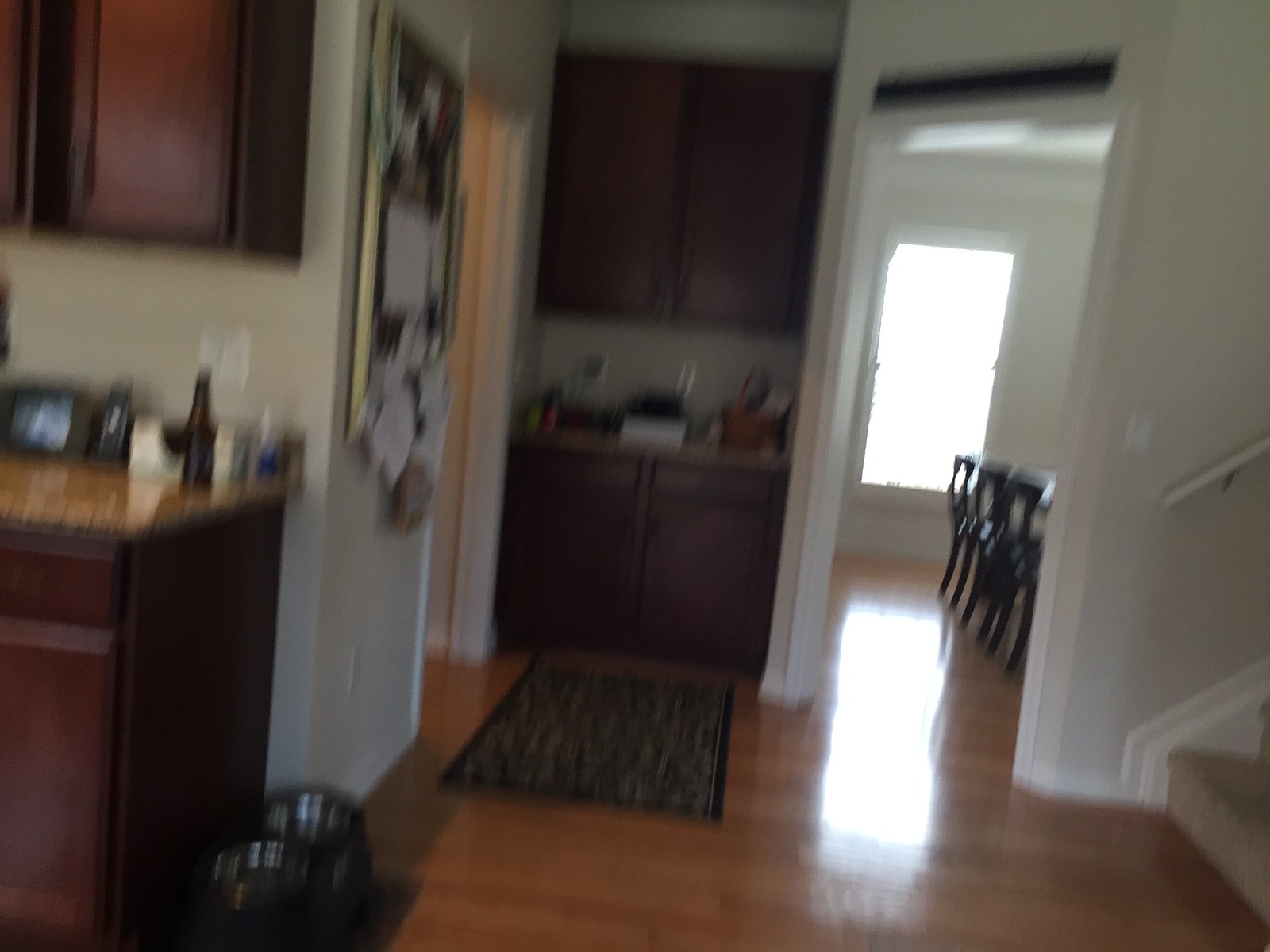The image depicts a cozy 1990s-era kitchen. On the right-hand side, there is a stairwell with beige carpeting that extends down and meets a wall before transitioning into a door, whose destination is unspecified. The kitchen itself features a nostalgic built-in coffee bar with two brown cabinets and a countertop, though the image's blurriness prevents a clear view of the countertop's contents. Adjacent to the kitchen is an open doorway leading into the dining room, where a table with three chairs and a large window can be seen, inviting natural light into the space. Near the base of the stairs, there is a raised bowl, likely for a larger dog. The stairwell wall hosts a bulletin board cluttered with various papers, suggesting an organized yet busy household. The floors throughout are wooden, with a small area rug placed near the stairwell, adding a touch of warmth and comfort to the homey environment.